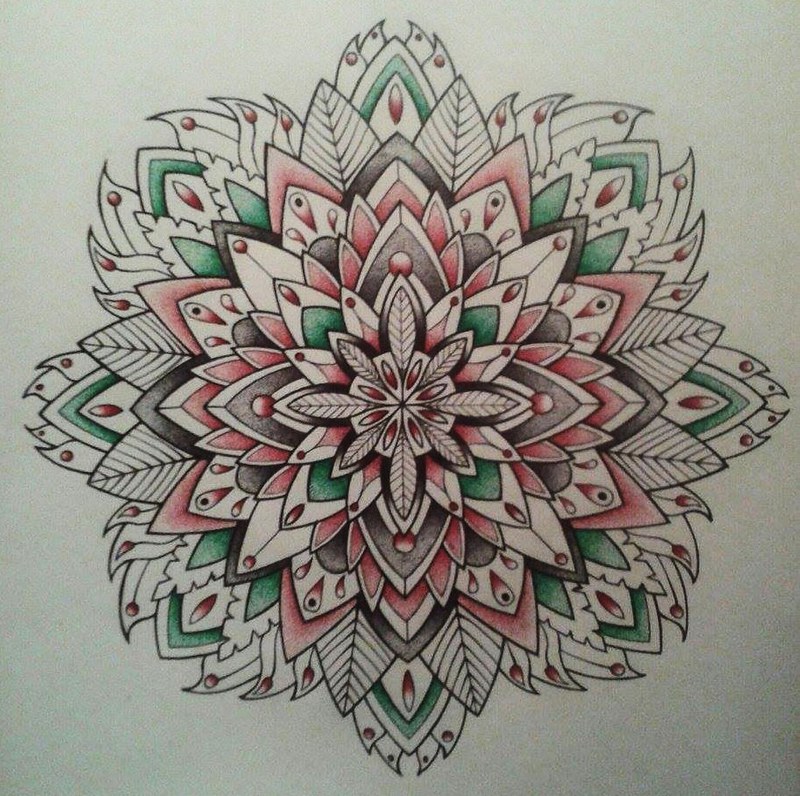This image features an intricate ink drawing on slightly off-white paper, showcasing a symmetrical design that exhibits a fascinating play of shapes and colors. At the heart of the composition lies a central circle, from which leaf-like shapes radiate uniformly in all directions. Each subsequent layer of the drawing mirrors this patterned emergence, creating a cohesive and balanced visual experience. The symmetry is precise, ensuring that if the design were folded either horizontally or vertically, each half would match perfectly. Various sections of the design are colored in vibrant hues: some leaves are adorned in green, others in red, with additional accents of black and light grays interspersed throughout, adding depth and complexity to the overall artwork.